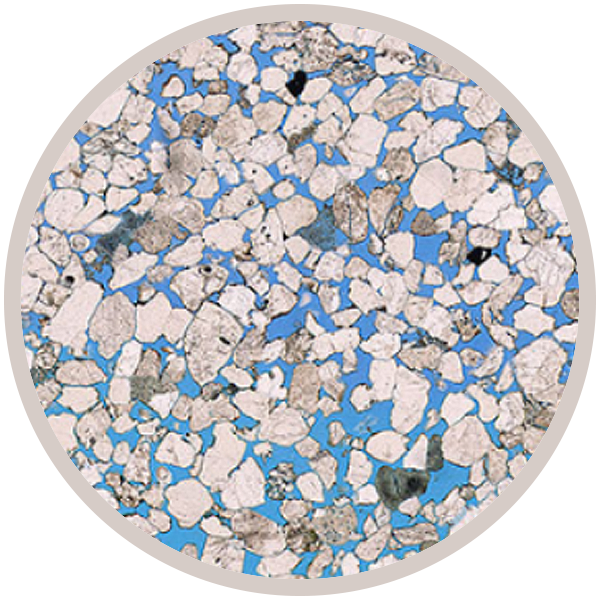The image depicts a circular object with a varied background and textures. The circle has a beige or gray border. Within the circle, the dominant background is a bright blue color scattered with non-uniform shapes that resemble stones or gravel. These shapes come in different shades, primarily white, accompanied by some gray and a few black or brown ones. Among these, certain shapes, like a very dark gray piece resembling an arrowhead and another akin to a piece of popped popcorn, stand out. The distribution of these shapes is random, creating an appearance that evokes both natural stone patterns and possibly, a stylized representation of landmasses scattered across a blue sea on a globe. The exact nature—whether a drawing or a depiction of stepping stones—is ambiguous, but the textured elements provide a visually intriguing, intricate pattern.